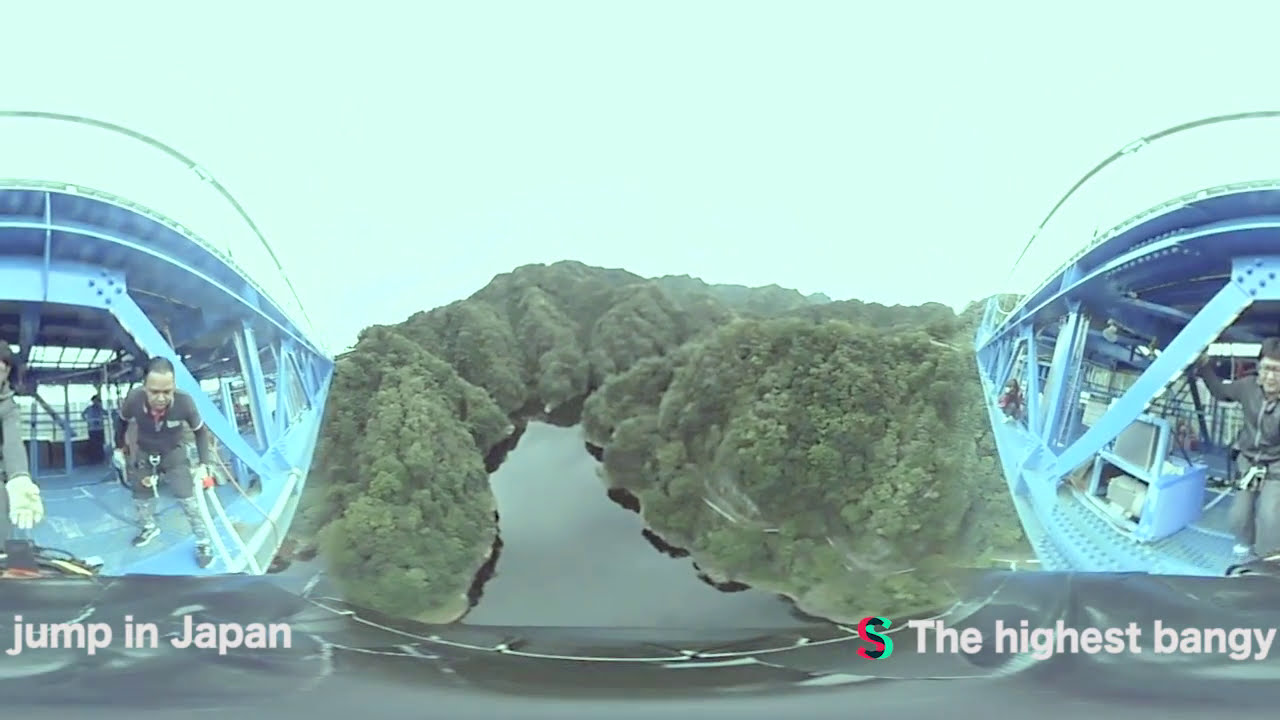The image is a panoramic graphical representation of a scenic valley in Japan, prominently featuring text at the bottom proclaiming, "Jump in Japan -- The Highest Bungee." In the center, a calm, flat lake forms an upright triangle shape with slightly curved top corners, encircled by lush green hills densely blanketed with tall trees, their branches hidden from view. The sky above is a muted blend of white and gray, creating a tranquil backdrop. To the left side of the image is an oversized letter 'S,' with its backside painted red and the front and right sides in green.

Flanking the valley on both the left and right sides are blue steel beam bridges extending from the background towards the foreground. Positioned on these bridges are individuals preparing for a thrilling bungee jump, ropes securely wrapped around their waists. Nearby, other people, likely crew members, assist the jumpers. A narrow path can be seen cutting through the bottom half of the right hill, emphasizing human interaction with this natural setting. This captivating scene highlights the excitement and adrenaline of bungee jumping from a high vantage point above the tree line.